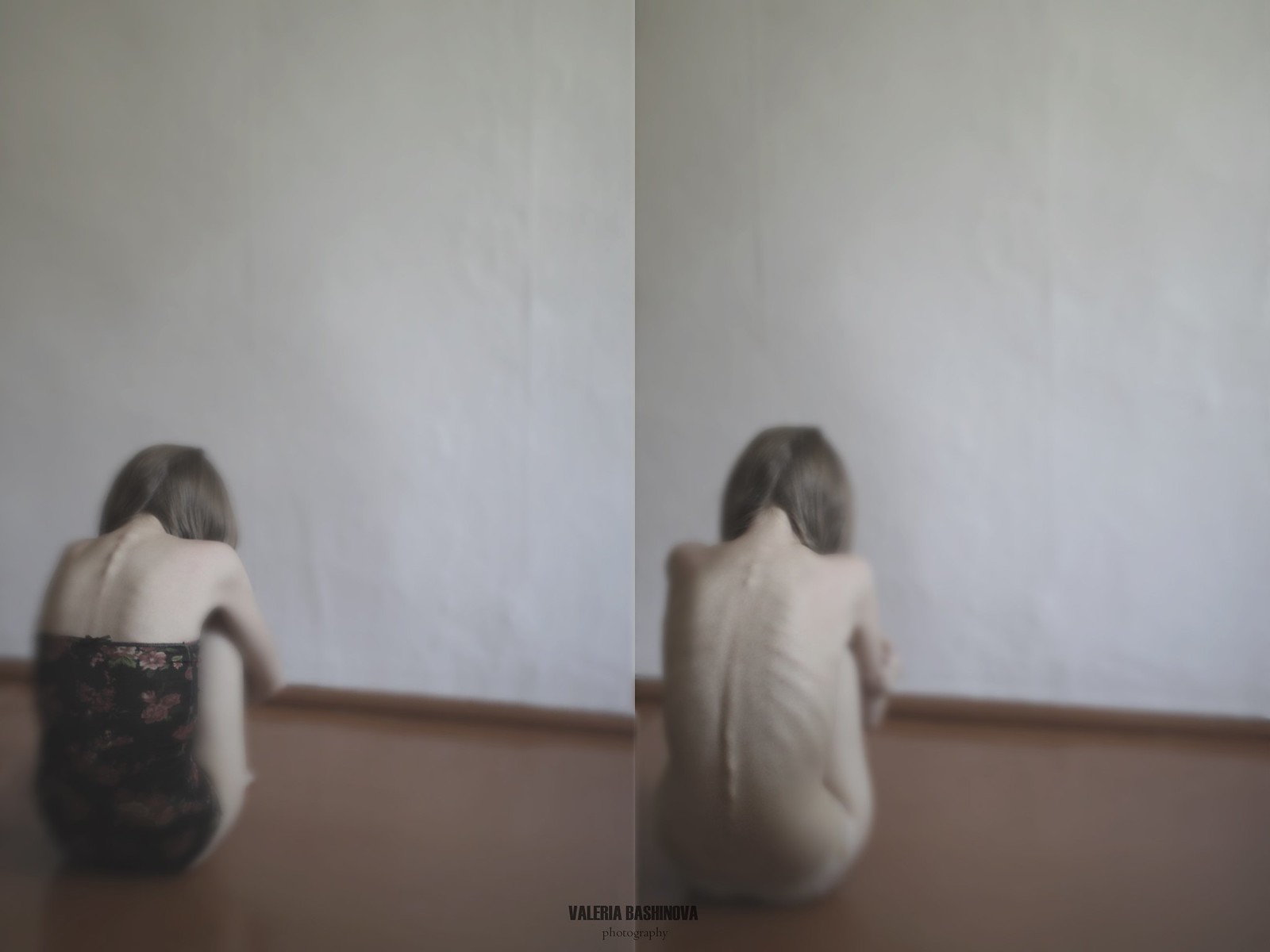The image features two side-by-side photographs by Valeria Byshinova Photography, overlaid with the photographer's name at the bottom. Both images depict the same woman sitting on a brown floor against a white wall, with her arms wrapped around her knees, and her head bowed, showcasing her spine prominently. In the left image, the woman is wearing black lingerie adorned with red flowers, and her light brown hair cascades down her back. In contrast, the right image presents the woman in the same pose but naked, accentuating the contours of her spine and ribs. The stark simplicity of the setting and the raw vulnerability of the woman's posture create a powerful visual narrative.